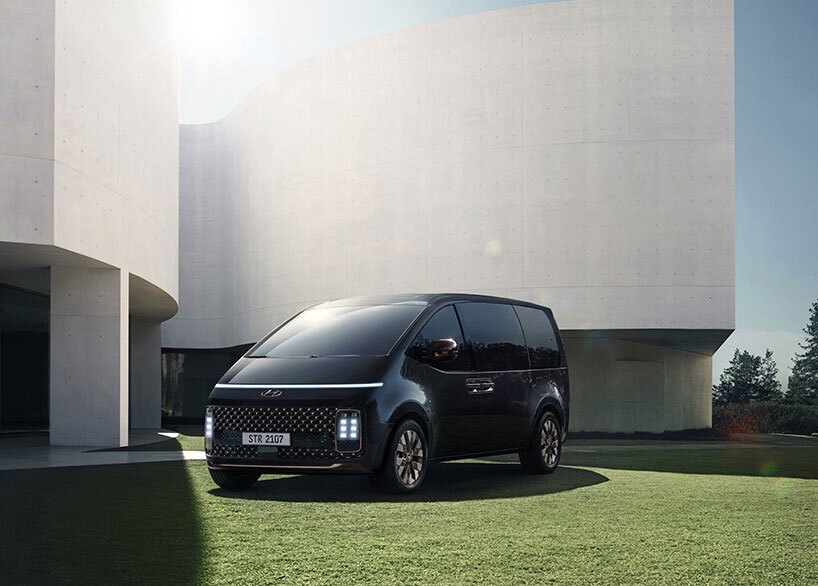This color photograph features a glossy black Hyundai Staria minivan, prominently centered, parked on manicured, verdant grass in front of a strikingly modern, curvy white concrete building. The building, reminiscent of a modern art sculpture, boasts large pillars and an intriguing, windowless design. The minivan, with its distinctive blacked-out windows and a European style white license plate reading "STR 2107," has a slanted front with a rounded end, LED headlights, and a black and gray grille. The sky above is a clear, vibrant blue, with a hint of conifer trees visible in the distance to the right. To the left, another part of the building features an entrance with a square door. The overall scene presents a juxtaposition between the futuristic vehicle and the minimalist, modern architecture, bathed in natural sunlight.